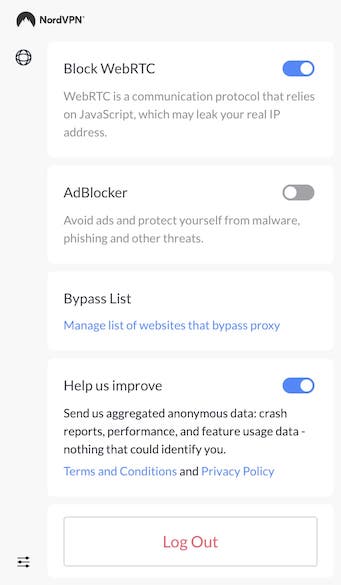This is a screenshot showcasing the settings menu in the NordVPN app, set against a light gray background. In the upper left corner, there's the NordVPN logo which features a semi-circle design, with the top half in black and the bottom half resembling a mountaintop. 

Below the logo, there is a white rectangular section with black text that reads "Block WebRTC," which has been toggled on. A description underneath explains that "WebRTC is a communication protocol that relies on JavaScript, which may leak your real IP address."

Following this, another white rectangle contains the text "Ad Blocker," which is toggled off. The accompanying description reads: "Avoid ads and protect yourself from malware, phishing, and other threats."

The next white rectangle in the sequence is labeled "Bypass List." Below this label is a clickable link that says "Manage a list of websites that bypass proxy."

Further down, another white rectangular section displays the text "Help Us Improve," with the toggle switched on. The descriptive text below states: "Send us aggregated anonymous data: crash reports, performance, and feature usage data—nothing that could identify you." Additionally, there are links provided for the Terms and Conditions and Privacy Policy.

At the bottom of the settings menu, a red button labeled "Log Out" stands out.